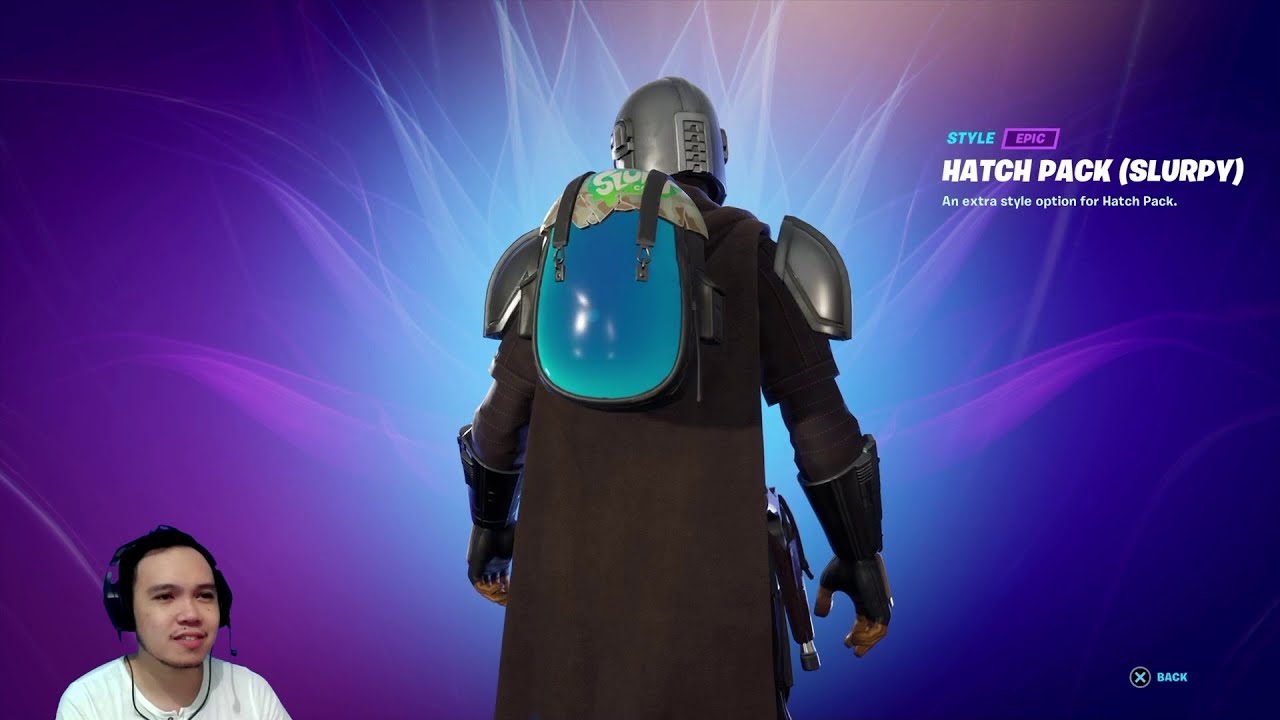The image is a detailed screenshot of a video game being streamed by a young man. Dominating the background is a mesmerizing blue and purple design resembling a lotus blossom, illuminated from its center with tendrils of light. At the center of this design stands a video game character, viewed from behind, donning a Mandalorian-style armored brown uniform complete with dark gray metal gauntlets, open-fingered gloves, and a metallic helmet. The character is also equipped with a distinct black and blue backpack, featuring green accents and white writing on the top, along with two metal straps over a blue stone center.

To the right of the character, text in various colors reads "Style," "Epic," "H-Pack (Slurpee)," and "Extra Style option for H-Pack." Additional interface elements include a circle with an 'X' and the word "Back" in the bottom right corner. In the lower left corner, a webcam feed shows the streamer himself— a young man with facial hair, wearing a white t-shirt and over-the-ear headphones with a microphone. He appears focused, slightly smiling, and is angled towards his left.